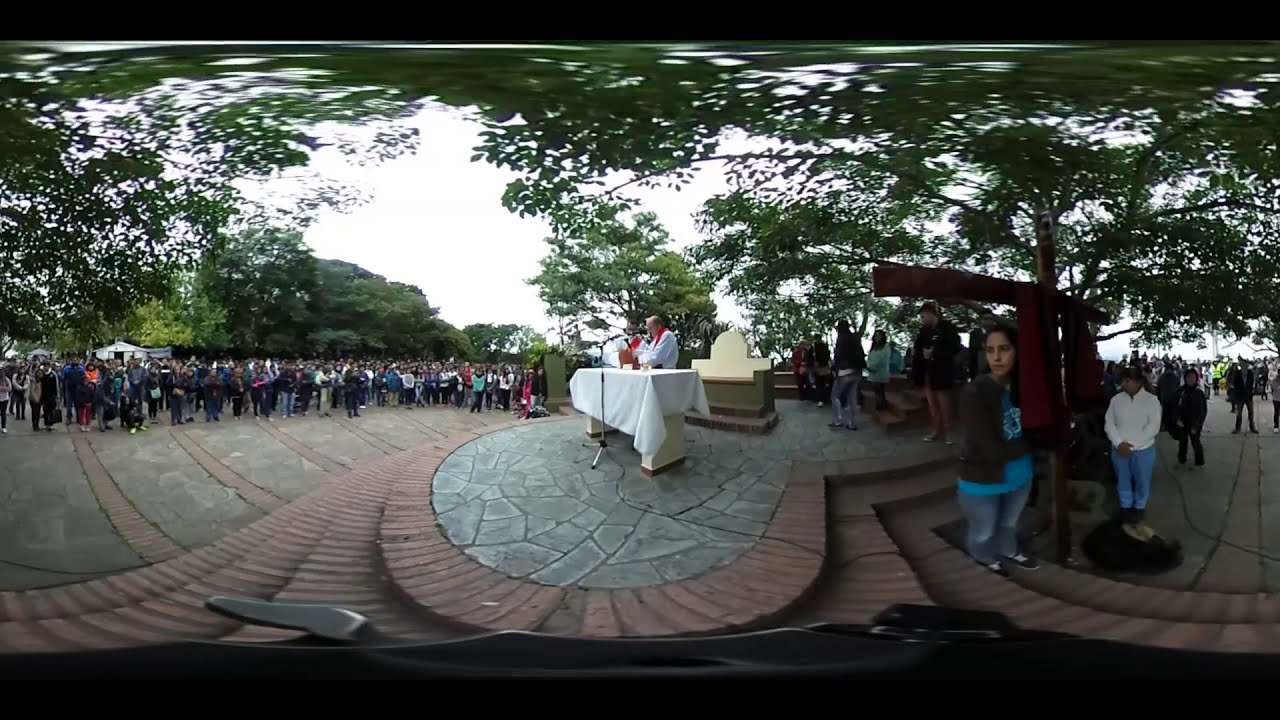The image depicts a panoramic, fisheye photograph of a public outdoor event, possibly an outdoor church service, taking place on an overcast day in a park. At the center of the elevated concrete and brick platform, there is a rectangular table draped with a white tablecloth. Still behind the table are two men dressed in white robes with red accents, one of whom appears to be a church leader or priest. The priest is speaking into a microphone placed at the podium. To the right, a woman in a turquoise blue shirt stands near a brown wooden cross. Surrounding the platform is a large crowd of people, densely gathered particularly on the left side of the image, showing hundreds in attendance. In the background, the warped fisheye effect accentuates the lush green tree branches that blend into the overcast sky. These elements collectively suggest a large, socially-distanced religious gathering, possibly from the early days of the COVID-19 pandemic.